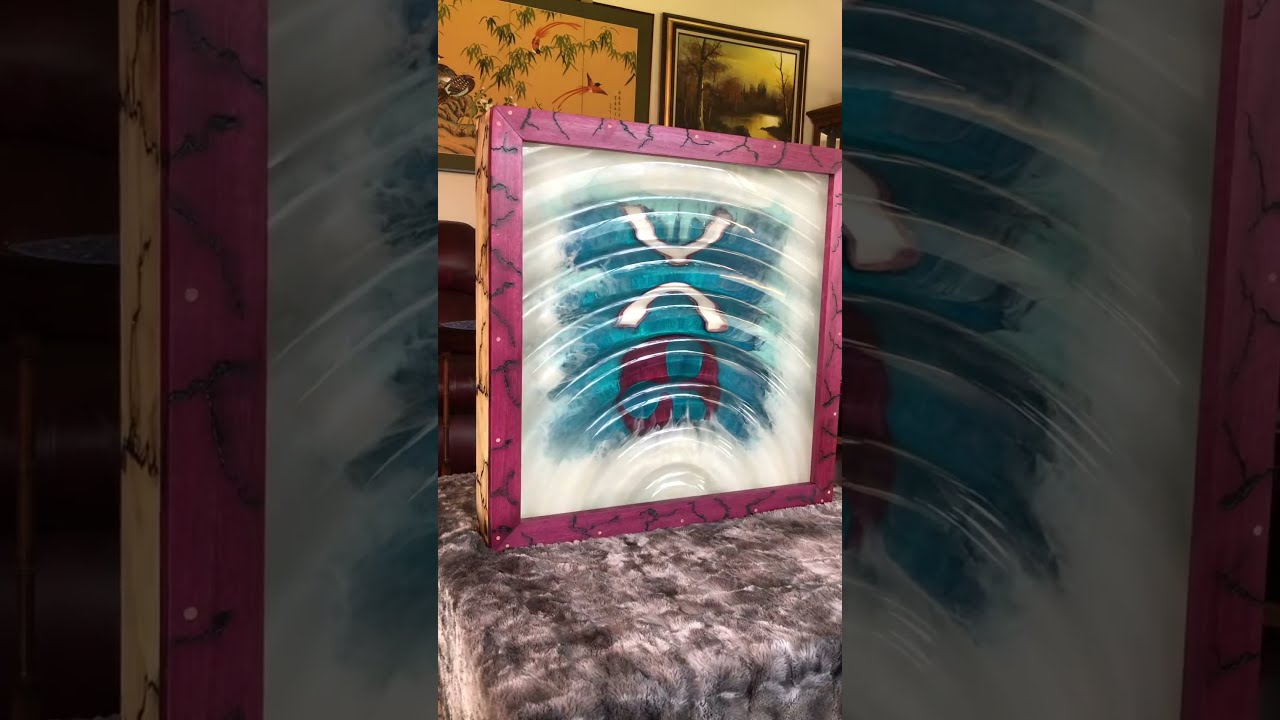The image depicts a photograph taken from a smartphone, showing a piece of artwork prominently displayed in a magenta-pink frame, resting on what appears to be a black and white marble table or stool. The artwork itself features a white background with blue and white brushstrokes forming ripple-like patterns. At the center, there's a distinctive white "U" shape with an inverted "U" beneath it, creating a combined symbol. Below this, a red square encloses three blue circles, resembling a hazmat symbol. The background of the photograph includes a lighter gray wall adorned with two other pieces of art. On the right, a framed picture depicts a serene lake scene with tall trees and a golden dawn sky. To the left, another black-framed artwork shows tree branches against a yellow background, possibly featuring a butterfly. The topmost part of the primary artwork hints at an abstract cityscape. Overall, the composition blends abstract and natural elements, highlighted by varying shades of blue, white, and red, set against complementary teal and gray tones.